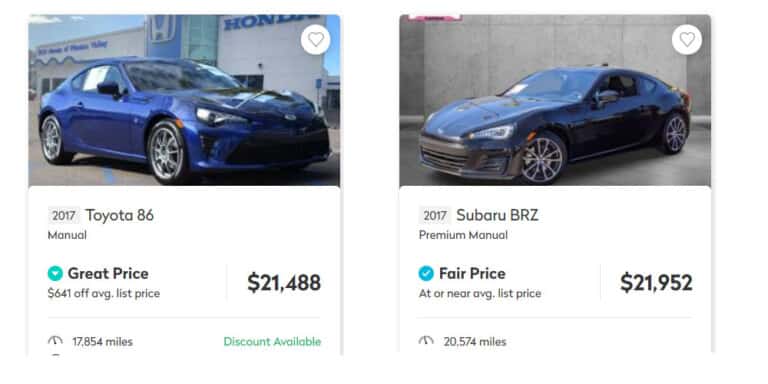The image is a side-by-side comparison of two sports cars, separated by a thin white border. 

**Left Side:**
- The top half features a blue sports car, slightly turned toward the camera, and facing right.
- In the background, there is a Honda dealership with gray walls and a blue section protruding out, displaying a large gray Honda emblem.
- A bit of the blue sky can be seen on both the left and right edges.
- In the top-right corner, there's a white circle with a white heart outlined in blue.
- Below this circle, there's text on a white background:
  - Top left in black lettering: "2017 Toyota 86"
  - Below that: "Manual"
  - A blue circle with a white check mark, accompanied by bold black text: "Great Price"
  - Subtext: "$641 off average list price"
- On the right side, large bold text states "$21,488" and below this, in blue, "Discount available."
- In the bottom left corner, just off the screen, the mileage of the car is mentioned.

**Right Side:**
- The image depicts a black sports car facing left, positioned outside a large gray wall and resting on a concrete surface.
- In the top right corner, the same circle with a heart is present.
- Below the car, on a white background:
  - Black text reads: "2007 Subaru BRZ"
  - Below that: "Premium Manual"
  - A blue circle with a white check mark, paired with bold black text: "Fair Price"
  - Subtext: "At or near average list price"
- On the right side, large bold text displays "$21,952."
- In the bottom left corner, just off the screen, the mileage of the car is mentioned.